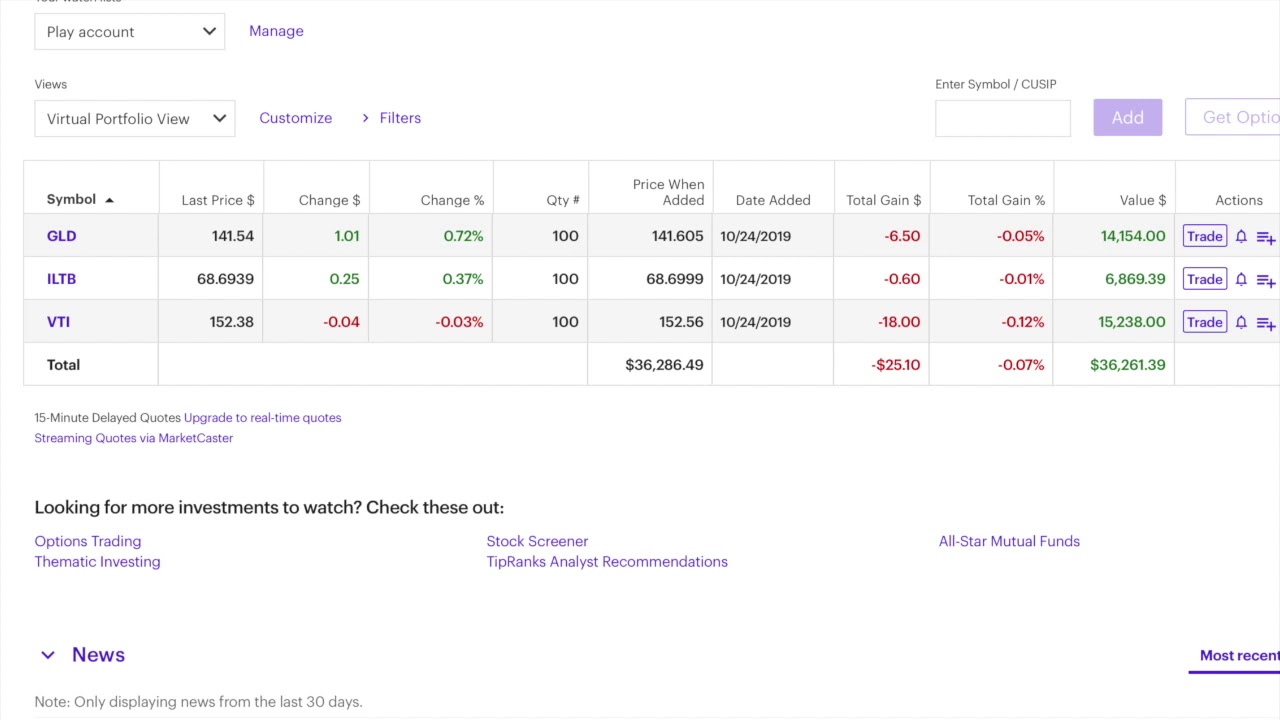This image is a cropped screenshot from a financial management website interface. It prominently features a white background in the top left corner with various interactive elements and navigational tabs.

At the top, there is a white search tab with a light gray border labeled "play account," accompanied by a dropdown menu. Adjacent to this in purple is the text "manage." Directly beneath it, in black, the word "views" appears, with another dropdown menu labeled "view" or "virtual portfolio view." To the right of this is a purple "customize" button. Continuing to the right is a greater-than sign (>) followed by the word "filters."

In the upper right section, there is a small, gray-bordered square with the phrase "enter symbol or /custom." To its immediate right is a purple tab labeled "add" in white text, and extending off the right side of the screenshot is a purple-outlined tab that says "get OPTIA."

Below these navigation elements is a detailed table with column headers including: "symbol," "last price," "change," "change percent," "quantity," "price when added," "date added," "total gain," "total gain percentage," "value ($)," and "actions." Each column is separated by vertical and horizontal lines. The table entries under "symbol" feature "GLD," "ILTB," and "VTI," highlighted in purple, and are followed by respective data such as numbers, dates, and percentages. At the bottom of the table, there are aggregated totals for specific columns like "price when added," "total gain," "total gain percentage," and "value."

Beneath the table, there are two brief purple lines followed by bolded text reading "looking for more investments to watch? Check these out." The interface presents additional recommendations arranged with two on the left, two in the middle, and one on the right side.

In the bottom left corner, there is a section labeled "news" in purple with a dropdown menu, and beneath it, in small black text, is a note stating "only displaying news from the past 30 days." On the right side of this section, the word "most recent" is underlined in purple.